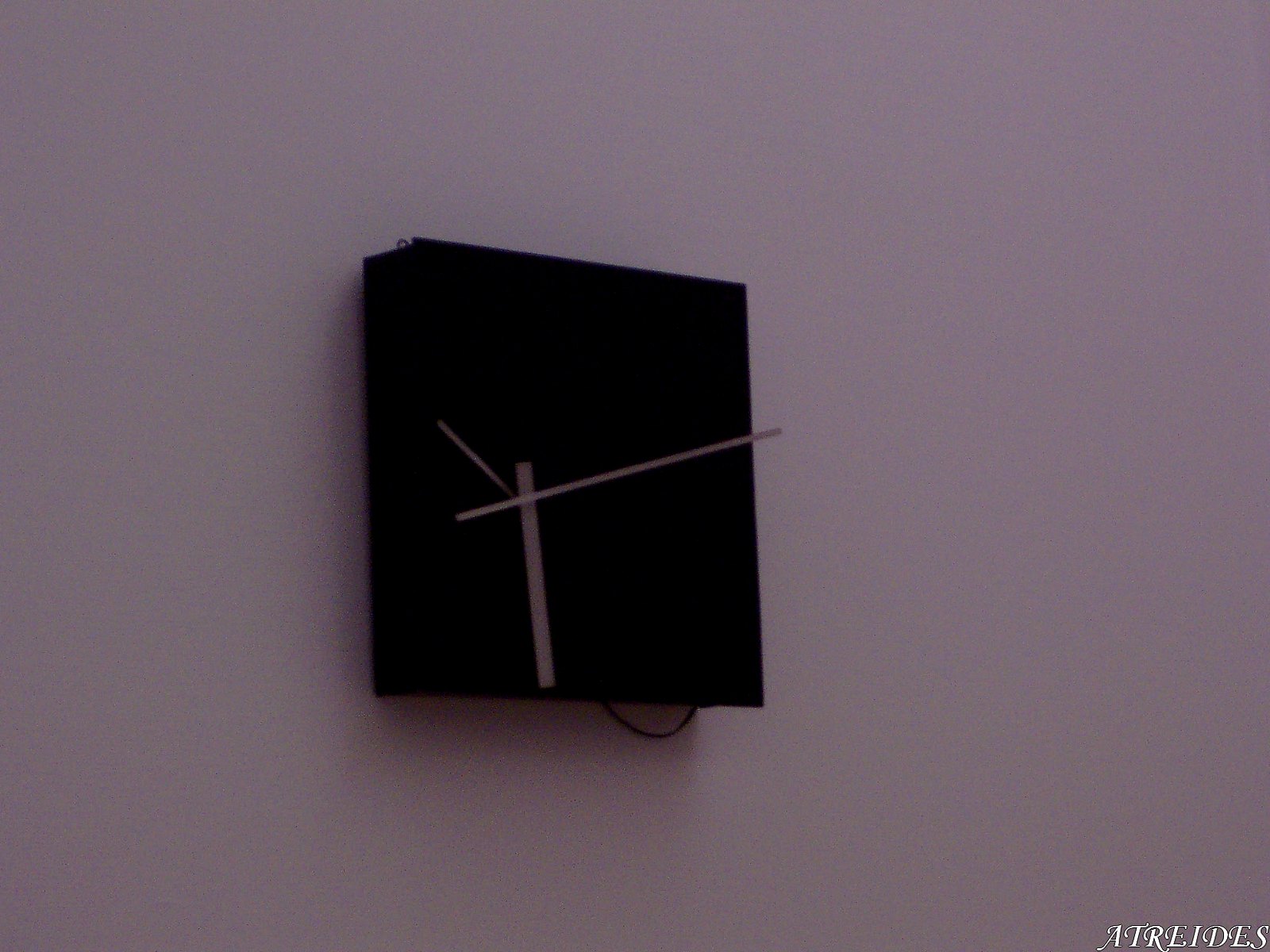This image features a modern, simplistic black box clock mounted on a pink wall, creating a striking contrast. The clock, resembling a piece of art, is square and thick with three exposed, silver clock hands that are positioned slightly left of center. The minute and second hands extend toward the right, with the hour hand pointing to the top left. A black cable cord can be seen hanging from the bottom right of the clock. Additionally, white text reading "Atreides" is inscribed in a fancy font on the bottom right of the image.